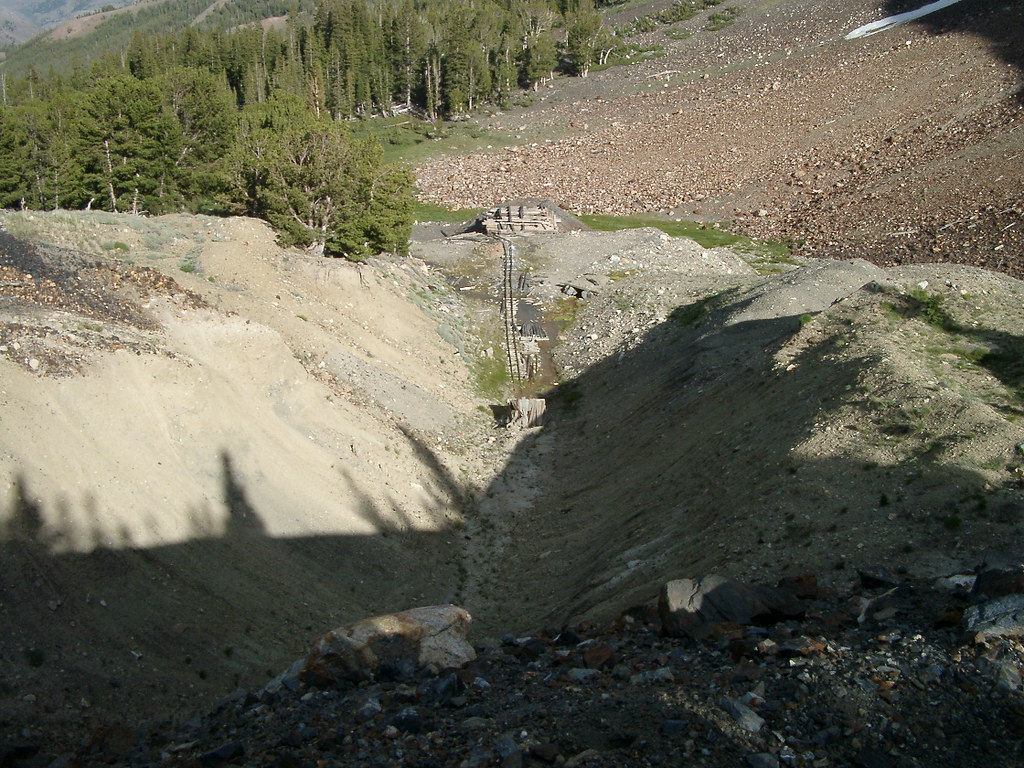This detailed photograph captures an expansive, rugged landscape as seen from the top of a mountain. In the foreground, rocky and gravelly terrain dominates, characterized by black rock and sandy, eroded surfaces. The center of the frame features a single railroad track emerging from a tunnel, running straight before curving off slightly, without any visible train. This track appears to cut through the valley that runs across the middle of the image, flanked by mountainsides on both the left and right.

On the top right, there's an open, gravel-covered space that contrasts with the lush pine trees densely populating the top left corner, indicating the diversity of terrain within the area. Further to the left in the background, the landscape transforms into a forested mountain vista with dark green pine trees. This natural setting suggests an old quarry now reclaimed by nature, providing a stark, yet harmonious, blend of raw, eroded surfaces and revitalized greenery, all bathed in selective sunlight that illuminates the middle of the photograph while leaving the foreground in shadow. No human presence is evident, enhancing the feeling of serene isolation.